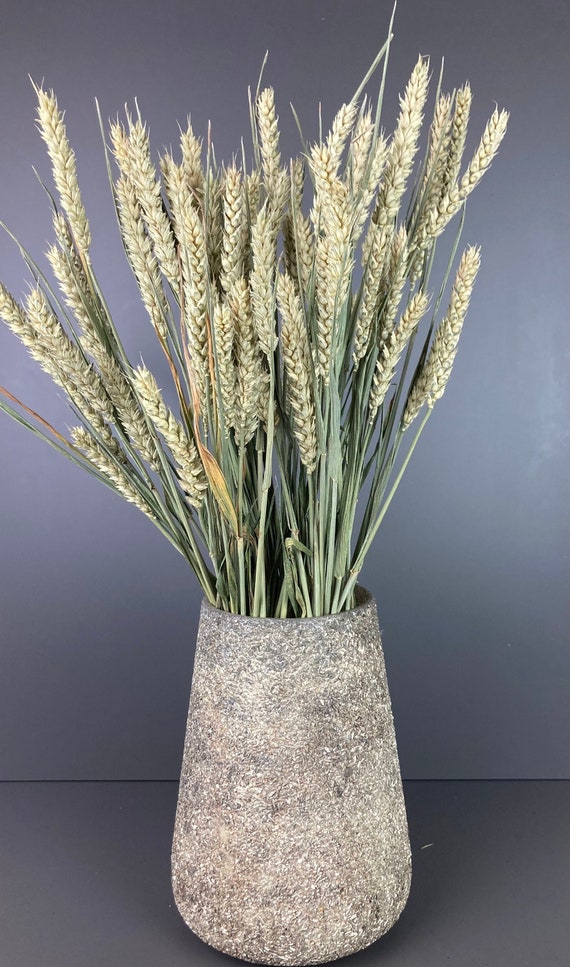This photograph features a textured, earthenware vase made of rough pottery in shades of brown, gray, and speckled with some white. The vase, which resembles a handmade piece, sits on a neutral gray background with a subtle gradient effect. The backdrop shows a clear delineation between the wall and the floor, marked by a thin black line. Inside the vase is a substantial bunch of wheat stalks, approximately 16 inches long, with the top 8 to 12 inches visible. The wheat has green stems and the characteristic yellowish tufts at the top. The light source accentuates the middle section, casting a gentle illumination on the wheat, creating a balanced and serene composition. The overall scene is reminiscent of a desolate plain, adding a natural and rustic ambiance to the image.